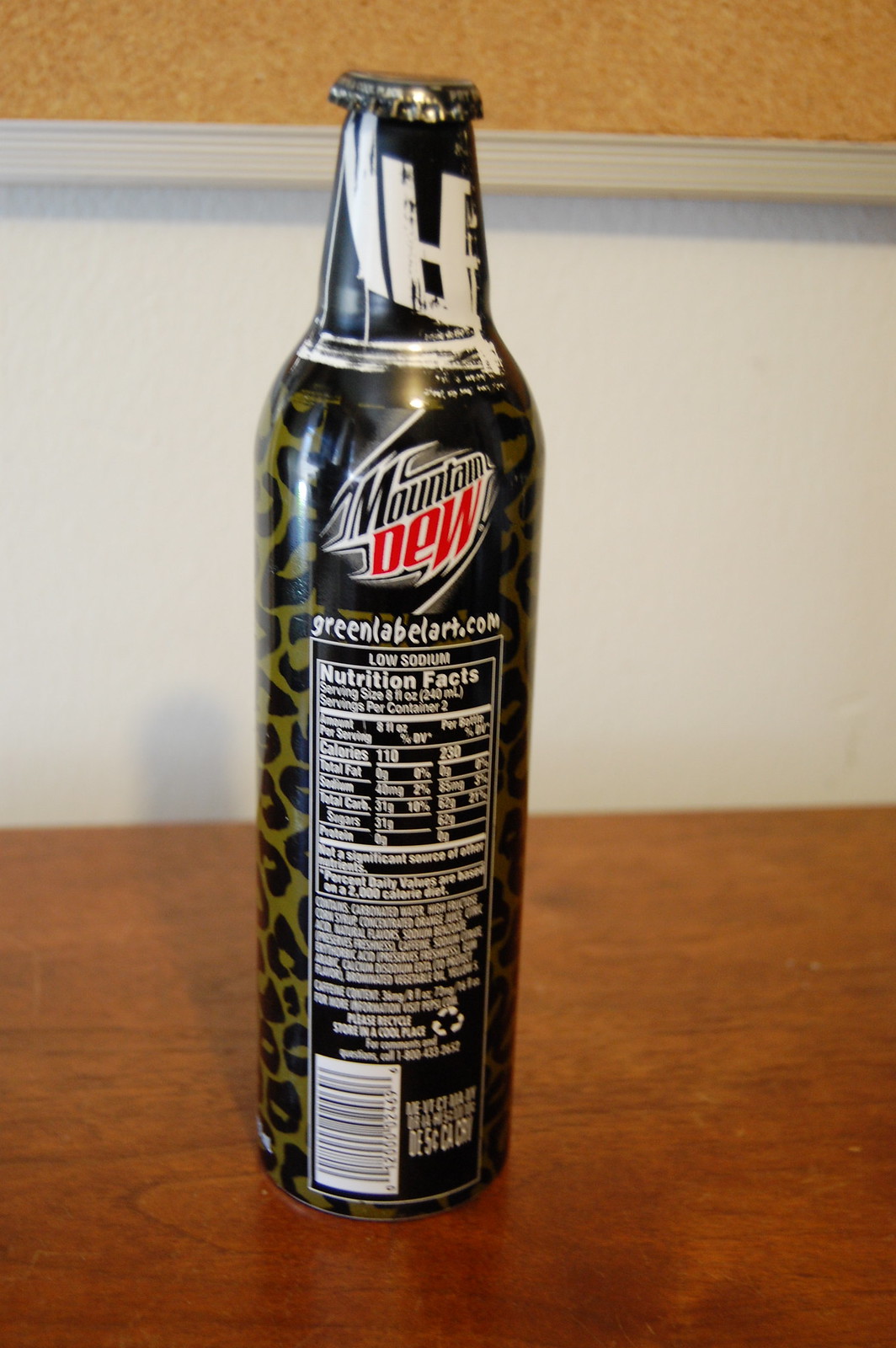This photograph showcases a distinct bottle of Mountain Dew placed on a medium brown wooden table. The background features a white wall and a cork board framed in white or tan, adding a subtle texture to the scene. The bottle, which appears to be either plastic or glass, sports a tapered neck and a pop-top metal cap that requires an opener. Its label exhibits a striking dark greenish-yellow and black leopard print design. Prominently displayed at the top is the iconic Mountain Dew logo with the text "Green Lab" followed by "label art dot com". Below the logo, in a white rectangle, are the nutrition facts listing low sodium among other details. The bottle's shadow is cast on the wall, further enriching the visual depth of the photograph.